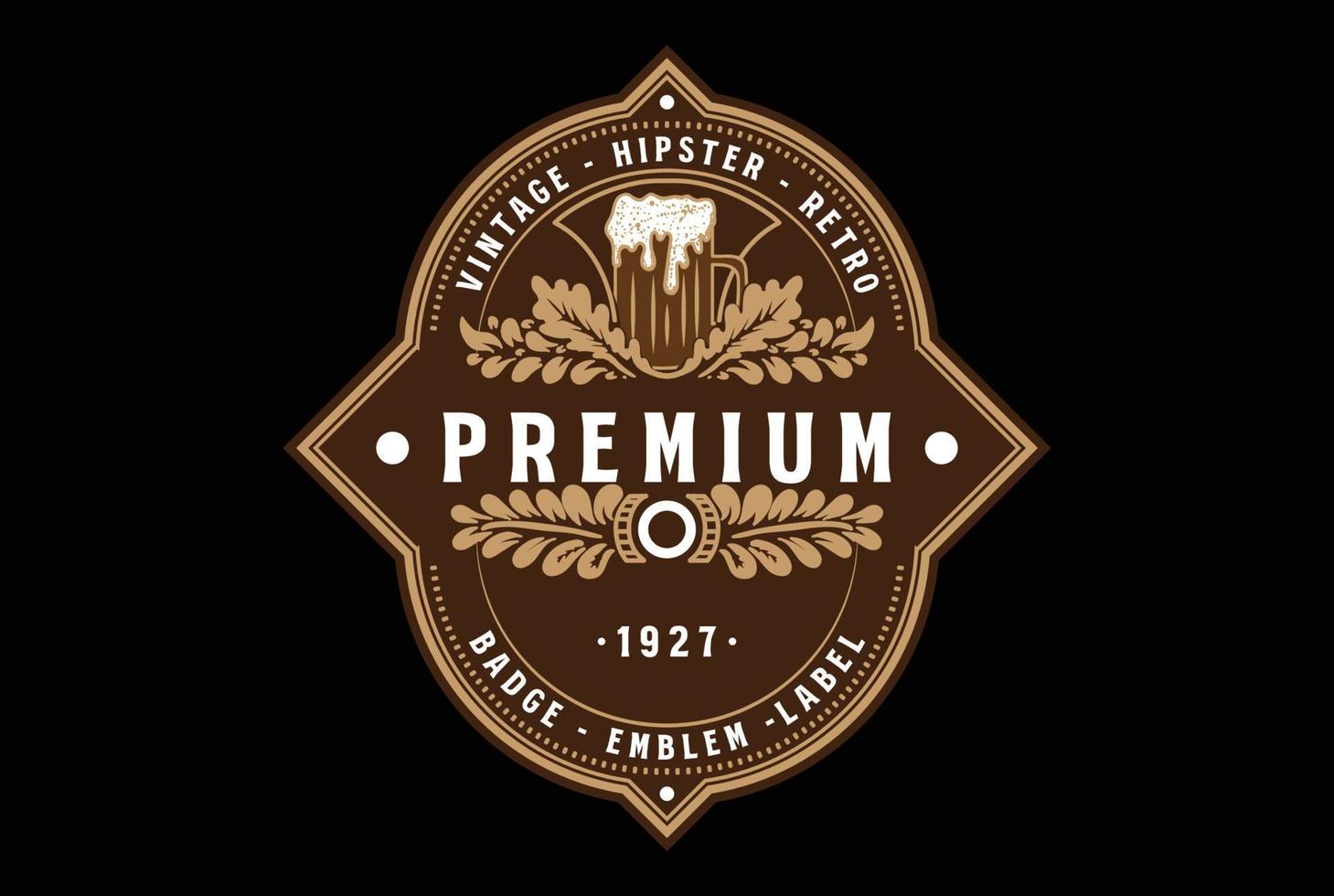The image showcases an up-close view of a vintage, hipster, retro-themed beer brand logo set against a completely black background. The logo, which has a brown, leather-like texture, is an oval shape with four distinct triangular points positioned at the top, bottom, left, and right—each point featuring a white dot. Along the top edge, the white text reads "Vintage," "Hipster," and "Retro" in a curved arrangement. Below this, there is a depiction of a frothy beer mug set against a cluster of brown leaves, likely representing hops. Central to the design, "Premium" is boldly displayed in large white letters. Directly beneath "Premium," the year "1927" is flanked by white dots, sitting above a circular motif with leaves extending from either side. Towards the bottom, the text "Badge," "Emblem," and "Label" curves along the edge in white. The entire logo is bordered by a lighter brown outline, enhancing its vintage appearance.